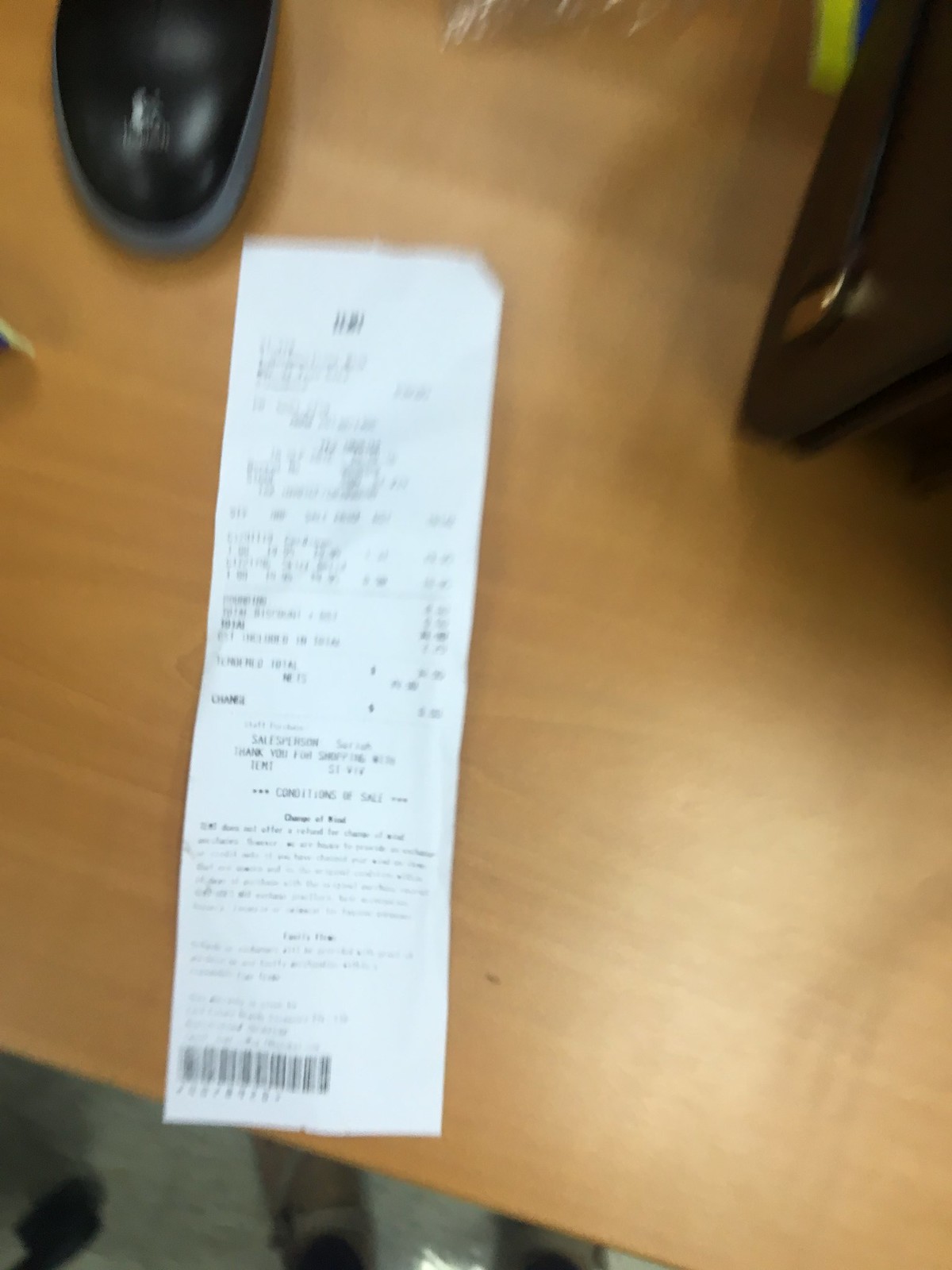An overhead photograph captures a light-stained, smooth wooden table. Prominently displayed on the table is a crinkled, elongated receipt, though the print is too blurry and distant to decipher. In close proximity to the receipt is the shiny toe of a polished black shoe. Adjacent to this, there is an indistinct black device or object. On the other side of the receipt, a portion of the gray floor beneath the table is visible. Two pairs of feet can be seen: one clad in light brown shoes, and the other foot to the left, donning a dark black shoe.